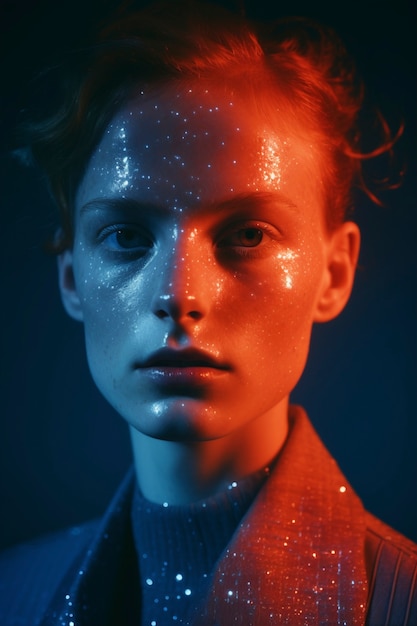The image presents a highly stylized and artistic nighttime portrait of a woman set against a transitioning background that fades from dark black at the top to lighter blue towards the bottom. The woman, with red hair styled up and pulled back, stands prominently in the frame. Her skin, luminous with glitter, displays a striking contrast: the left side of her face is dark while the right side is well-lit, revealing her natural skin tone. This light on her right side shifts between purple and red hues, adding a glossy effect to her appearance. Her serious, direct gaze and illuminated eyes draw immediate attention. She wears a turtleneck and blazer, both adorned with the same glitter that speckles her face, creating a cohesive and shimmering ensemble. The background remains solid with no text present, ensuring full focus remains on the illuminated, glittering figure.